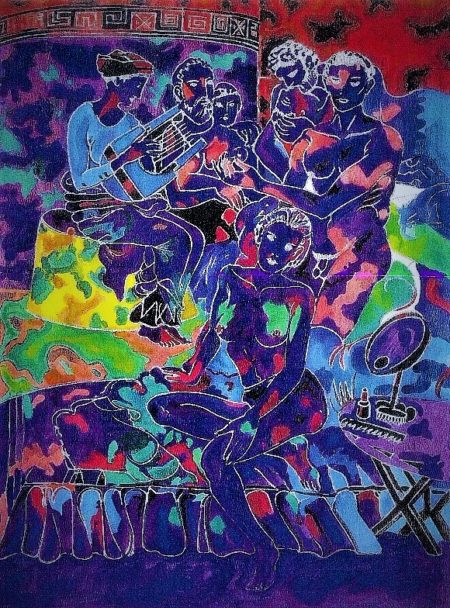The image is a psychedelic, multi-color artistic piece predominantly featuring shades of purple, blue, pink, and green. It is a vertically rectangular painting with no border or specific background. The central figure is a topless woman sitting on a bed, wearing black panties with green paint covering her breasts. Surrounding her are various individuals, including at least three other nude women and a nude man, evoking a Roman or Egyptian aesthetic. The background characters are painted in dark purple or dark blue, with some having white hair or wearing hats. One woman plays a lyre, a blue u-shaped stringed instrument with white strings, while other figures play horns and a drum. To the right of the central woman is a table holding a comb, a lamp or mirror, and what appears to be a bottle of nail polish. Bright greens and yellows illuminate the bottom left corner of the painting, and abstract text can be seen at the bottom of the image.